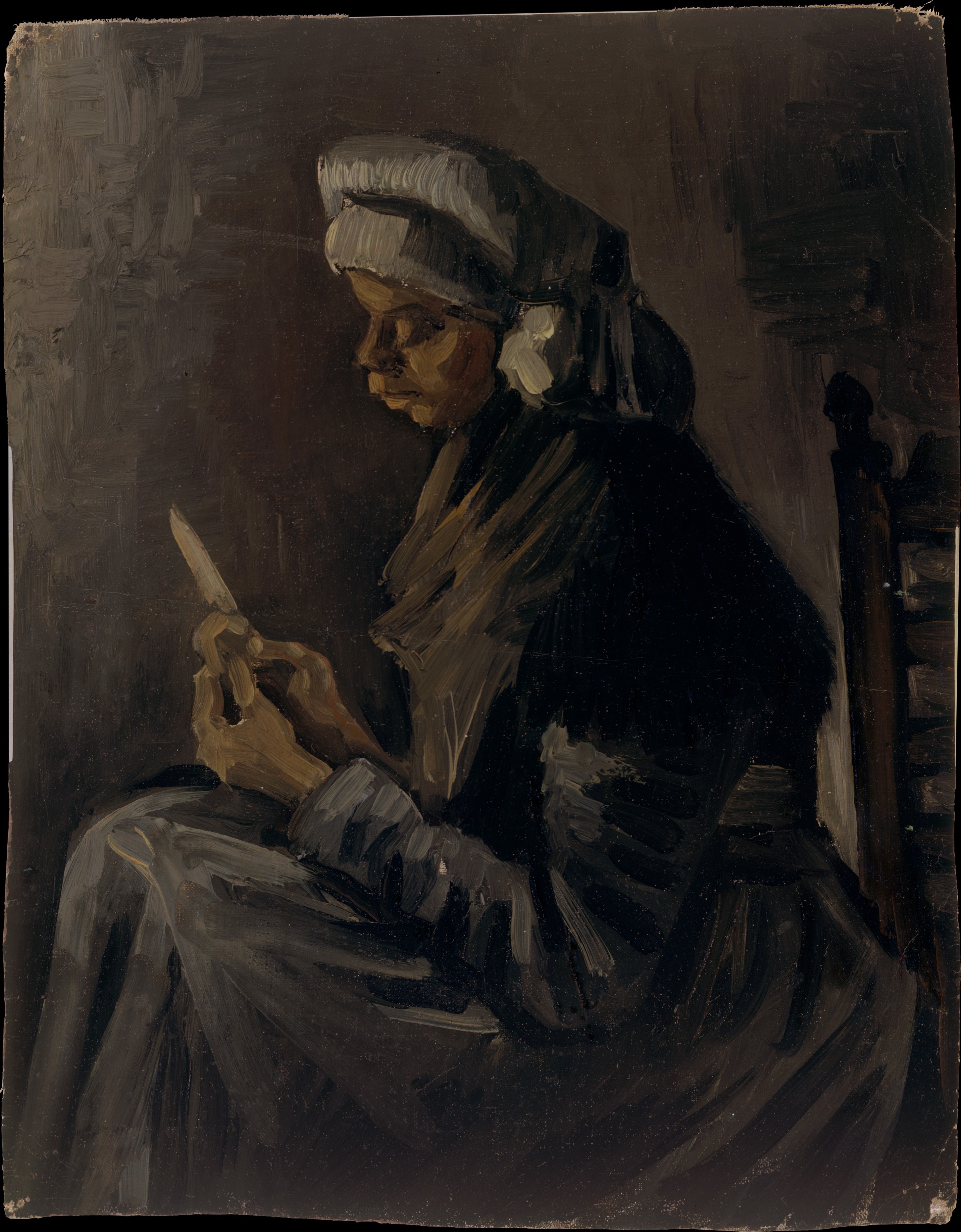The artwork appears to be an old, possibly frayed oil painting or postcard depicting an African-American woman from the late 1800s, characterized by broad brush strokes and a dark color palette. The woman, seen in profile and seated on a wooden chair facing left, is bent slightly forward, intently looking down at her hands. Her eyes are nearly closed as she appears to be engaged in an activity, perhaps whittling or reading, suggested by her holding a slender object and a knife. She is dressed in a long, thick, gray and black dress that covers her completely, with long sleeves extending to her hands. She also wears a large hat or cap adorned with a white tassel and might have white earrings. The overall muted gray background emphasizes the austerity and somberness of the scene, with the woman’s brown skin providing a stark contrast.